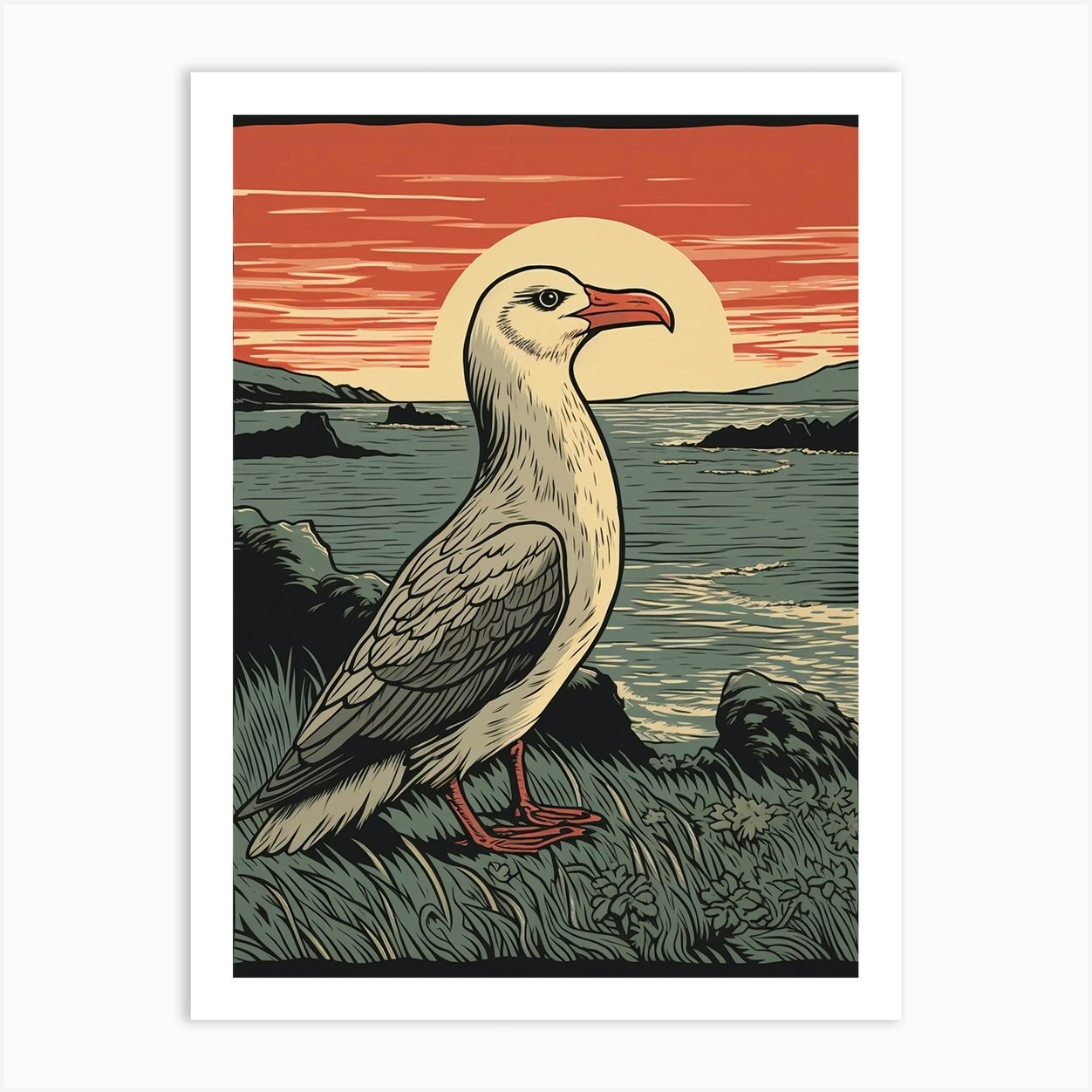The image depicts a highly detailed painting of a seashore bird, likely a seagull or duck, standing on muted green grass slightly blown by the wind. The bird faces rightwards, showcasing a white head with a black eye, a striking orange beak, and orange legs with webbed feet. Its body features a grey wing folded down against a whitish belly. Behind the bird, the land gives way to an expansive ocean, with visible white surf and silhouetted rocky outcroppings jutting from the water. The scene captures a dramatic sunset, with a semicircle of the yellow Sun setting into the horizon amidst a sky filled with red and yellow streaks. The overall palette of the painting beautifully balances shades of orange, grey, black, white, and tan, highlighting the bird's orange features and the glowing sunset.